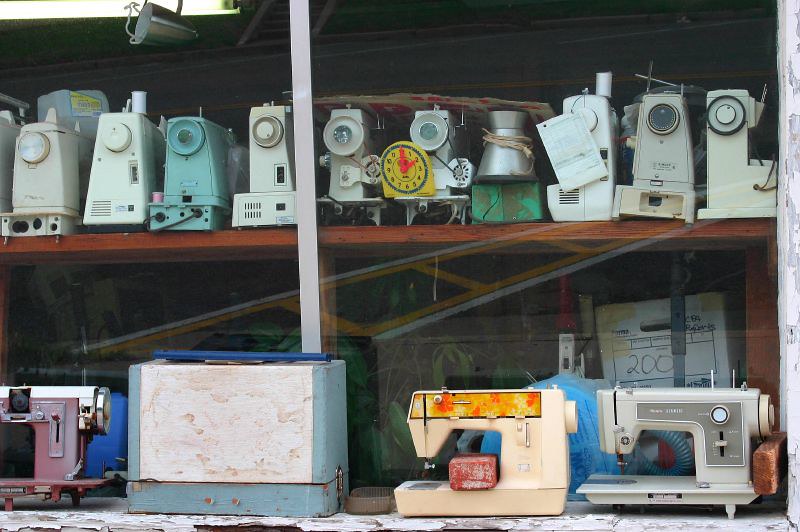This detailed photograph captures the storefront of an antique shop, possibly taken from an indoor perspective. The background features a wall that seems to be made of silver metal, with a wooden brown roof above it. The main focus of the image is on several shelving units in the foreground, constructed from lighter brown wood. These shelves are filled with an array of vintage sewing machines, all displayed side by side. 

The uppermost shelf prominently holds white sewing machines, each equipped with dials located on their sides or tops. The lower shelves display the sewing machines facing directly towards the viewer, revealing various levers and buttons, with the third machine on the right sporting a distinguishable yellow strip on its top. 

Nearly at the center of the top shelf, a conspicuous yellow and red school clock designed to teach children how to tell time is also visible. The sewing machines and the clock appear to be placed behind a glass pane, producing a reflection reminiscent of a roadway with white edges, yellow squares, and large black squares. 

In total, there are 12 sewing machines, varying in colors from basic white and beige to more distinct shades like gray, dark red, and light green. Additionally, there's a closed box on one of the tables, potentially containing another sewing machine. This collection of sewing machines appears to date back to the mid-20th century, with origins possibly spanning from the 1930s to the 1970s, showcasing their vintage aesthetic and historical value.